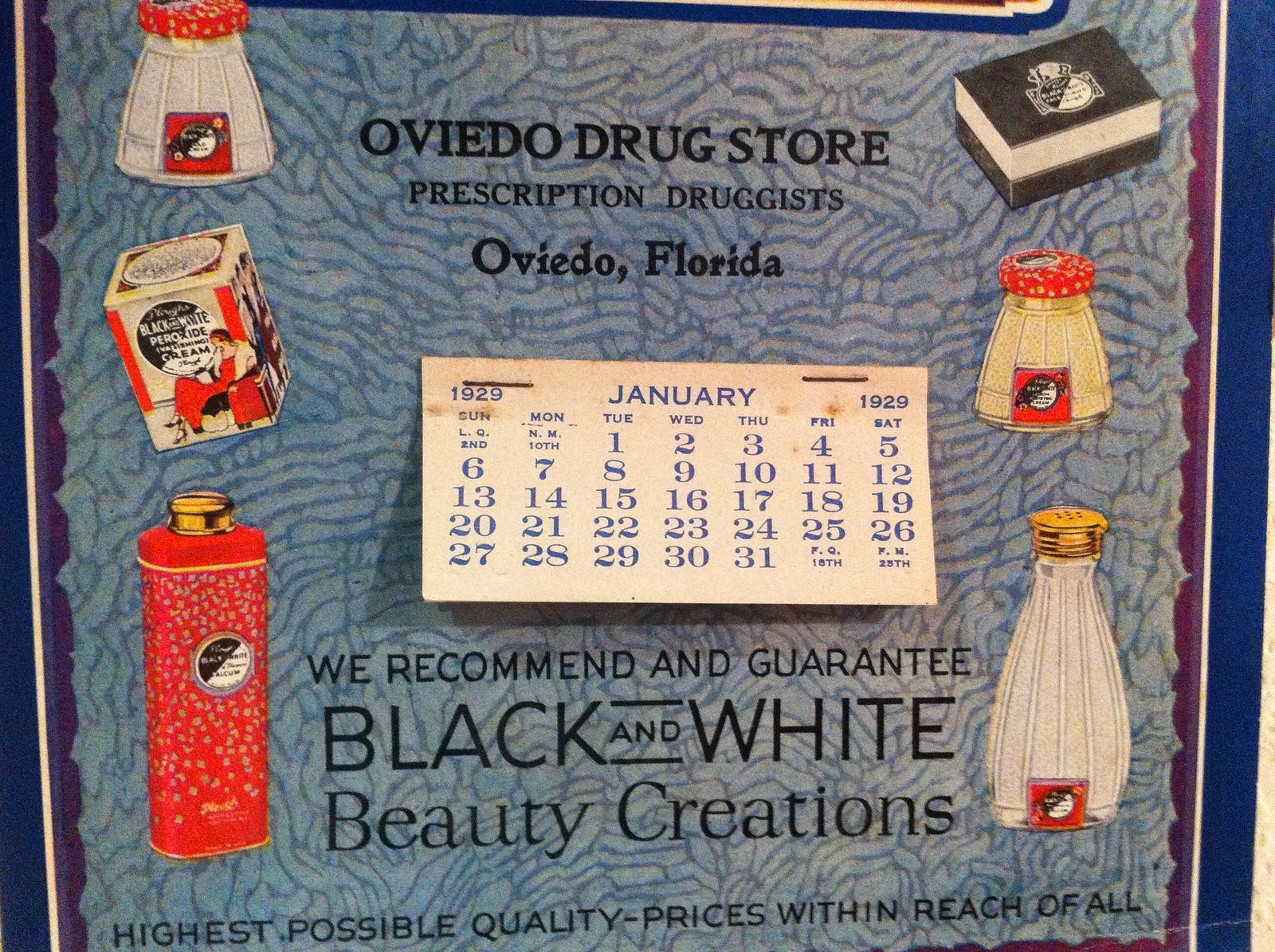This image captures a vintage advertising calendar from the Oviedo Drugstore in Oviedo, Florida, prominently featuring "Prescription Drugist" at the top. The calendar displays January 1929 in white with blue writing, stapled at the center against a decorative blue backdrop. Flanking the calendar on both the left and right sides are various pictures of bottles and containers, representing medications and health care supplies such as shampoos and creams. Below the calendar, the promotional text reads: "We recommend and guarantee Black and White Beauty Creations, highest possible quality prices within reach of all." The calendar's design and detailed product imagery highlight the drugstore's offerings and commitment to quality and affordability.